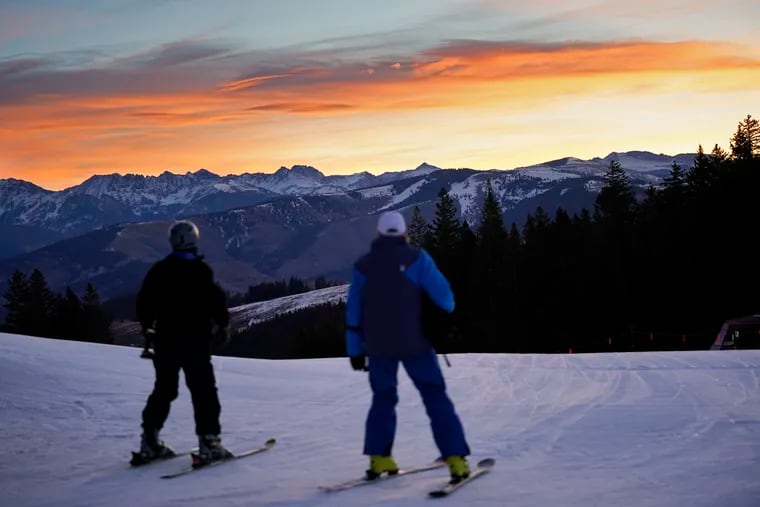This outdoor photograph, likely taken at dawn or dusk, captures two skiers atop a snow-covered mountain with their backs to the camera. They stand shoulder-to-shoulder, gazing out over a breathtaking, mountainous landscape. To the right, a skier is clad in a dark blue snowsuit featuring lighter blue sleeves and accented by yellow ski boots, perhaps wearing a white hat or helmet. The skier on the left wears an all-black ensemble, including a black helmet or hat and black ski boots. 

The expansive background reveals a stunning range of snow-capped mountains stretching from left to right, their bluish-gray peaks contrasting against the glowing horizon. The vivid sky transitions from bright yellows and golds at the horizon, through deep oranges, and into soft blues and grays at the upper edge of the image. Evergreens dot the landscape, prominently along the right side and into the middle ground, adding to the wintery scene.

Ski tracks suggest previous activity on the slope, though the skiers remain stationary, immersed in the serene beauty of the rising or setting sun. This spectacular blend of natural elements and the anticipation of a thrilling descent encapsulate the tranquil yet invigorating essence of alpine skiing.